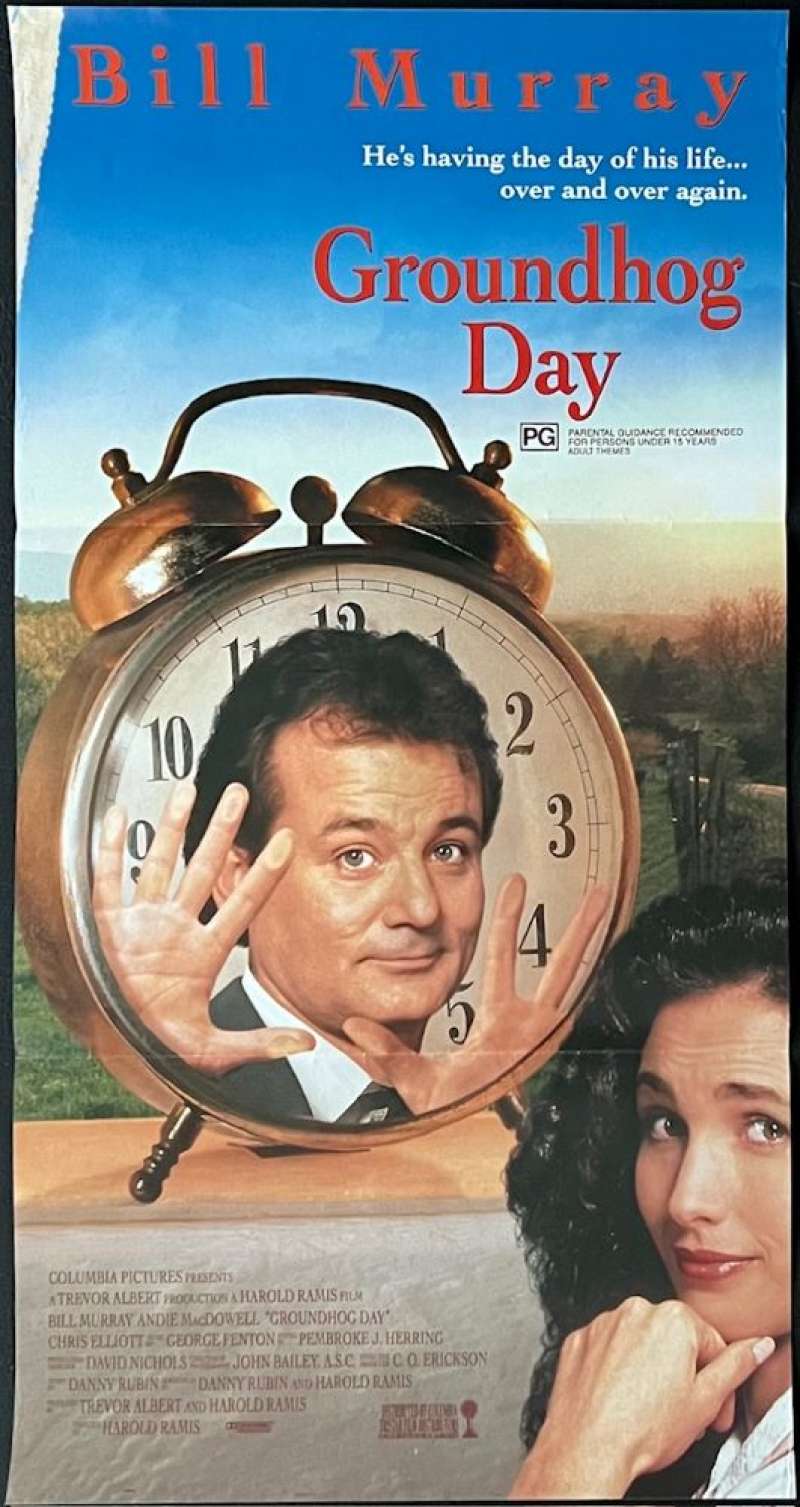This is a movie poster for the comedy film "Groundhog Day" starring Bill Murray and Andie MacDowell. The entire poster is enclosed by a thin, black frame. At the top, set against a blue sky background, Bill Murray's name is prominently displayed in red, spanning from left to right. Below his name, the tagline "He's having the day of his life over and over again" is written in white font, followed by the film's title "Groundhog Day" in red. Directly underneath is the PG rating logo with the advisory "Parental guidance recommended for persons under 15 years, adult themes."

Dominating the poster is a large, copper-colored wind-up alarm clock with a white face and black numbers. Bill Murray's face is superimposed on the clock, smiling slightly while appearing trapped behind its glass, with his hands pressed against it. He is dressed in a black suit coat and white shirt, looking directly at the viewer. To his right is Andie MacDowell, depicted with brown, curly hair, dark pink lipstick, and wearing a white shirt. She rests her chin thoughtfully on her left hand and gazes at the viewer.

The bottom half of the poster features extensive credits in red text, including "Columbia Pictures Presents," "A Trevor Albert Production," "A Harold Ramis Film," followed by the names of Bill Murray, Andie MacDowell, and other cast and crew members like Chris Elliott, George Fenton, Pembroke J. Herring, David Nichols, John Bailey ASC, C.O. Erickson, Danny Rubin, and Harold Ramis. Additional smaller text fills the rest of the credit block, concluding with more production details, although some of this text is too small to read clearly. In the bottom center, there's an unreadable block of text next to a small red circle set atop a post. The background scene behind all these elements includes a depiction of trees, grass, and an open sky, adding a natural outdoor ambiance to the poster.